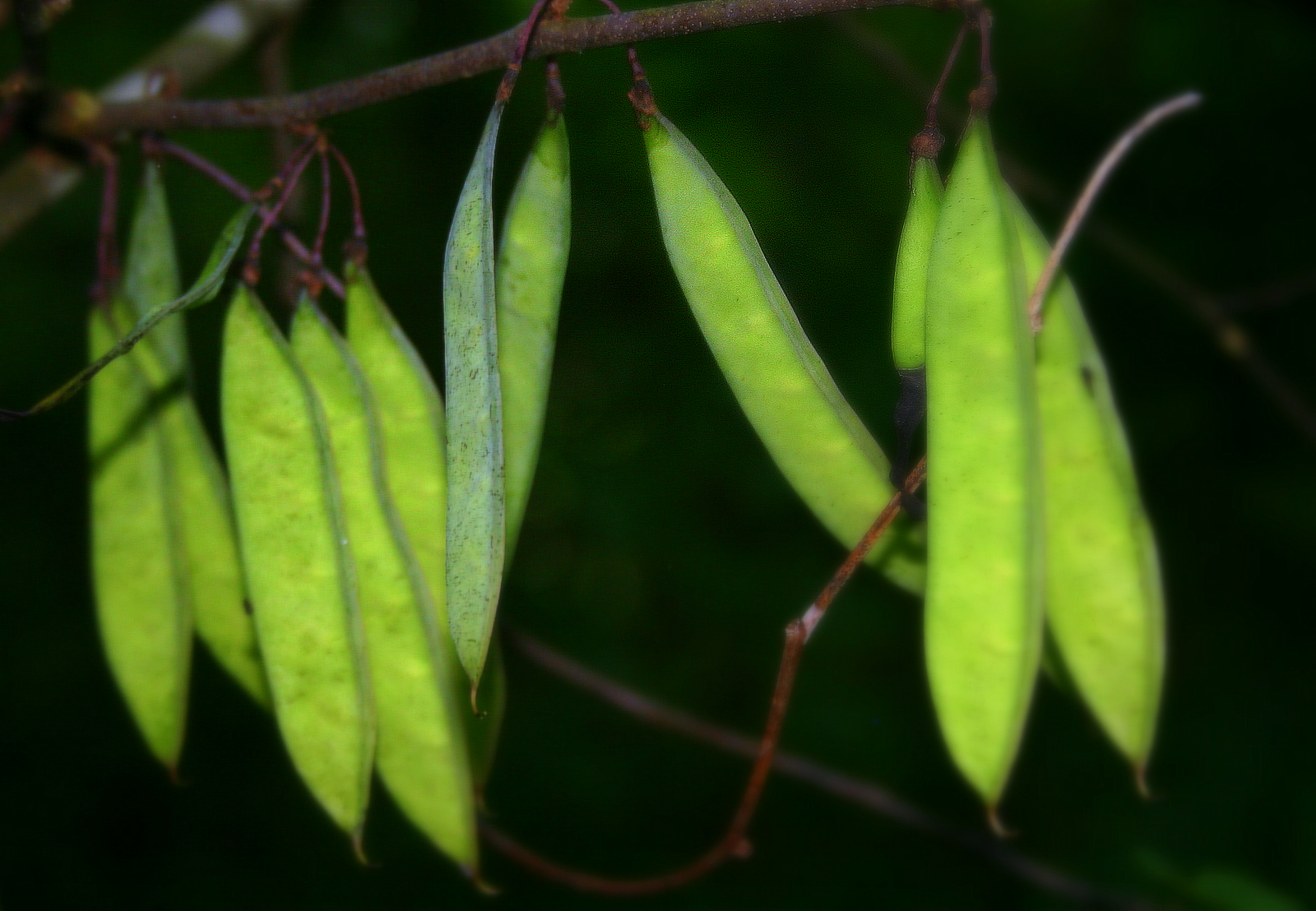The image showcases a botanical scene with a single diagonal branch stretching horizontally across the frame. Attached to this branch are several clusters of pea pods, reminiscent of sugar snap peas or snow peas, each hanging vertically from short stems. The pods, primarily green with a hint of yellowish tint, suggest they are not fully ripe. The reddish-purple color of the branch and stems contrasts against the dark, blurred greenery in the background. Lit by a flash, the peas are the focal point of the photograph, revealing the intricate details of their form and structure against the indistinct botanical backdrop.